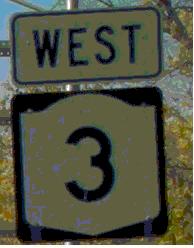A close-up photograph of a highway street sign is presented in this image, though its clarity is compromised by significant blurriness and noise, likely resulting from a high ISO camera setting. The top portion of the sign features a rectangular white and black marker displaying the direction "West." Beneath it, there is a square sign with a black border enclosing the number "3." This suggests the sign is for a highway or major road. The background is filled with indistinct tree branches and leaves, indicating a possibly autumnal setting, although the details are difficult to discern due to the image's tight framing and poor quality.